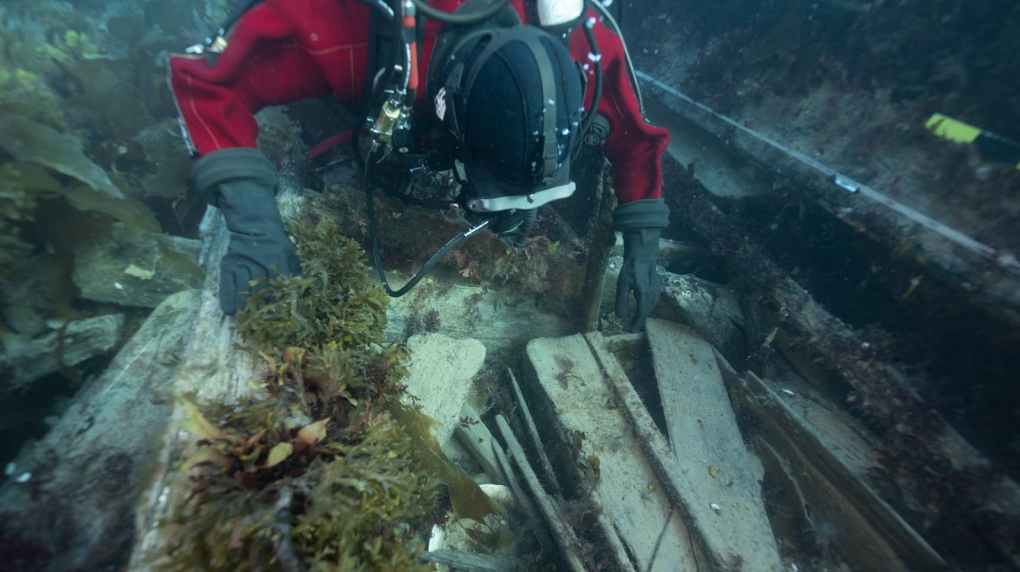The image depicts an underwater scene featuring a scuba diver examining what appears to be the remnants of a shipwreck. The diver is attired in a red scuba outfit, complemented by black gloves and a black headpiece. He is oriented head-down, closely inspecting the area beneath him. Surrounding him, there are bubbles rising from his headpiece, and air hoses extending from his helmet to his air tank. The underwater environment is dimly lit, but there are streaks of light penetrating the water, illuminating sections of the scene. The diver is focused on a collection of wreckage, primarily consisting of broken wooden planks interspersed with metal fragments. Notable green vegetation, such as seaweed, is entwined around the debris, particularly visible near the diver's right hand and behind his right arm. The right side of the image is darker and features long metal planks, suggesting the diver is exploring a shipwreck site.